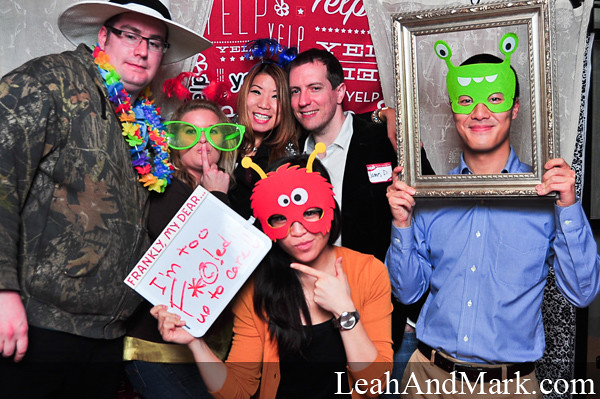This is a vibrant and casual group photo of six people at a Yelp event, indicated by the "Yelp" sign in various fonts in the background. The first person on the left is a man in a camouflage jacket, colorful Hawaiian lei, black and white wide-brimmed hat, and glasses. Next to him is a woman sporting oversized green sunglasses and red horns, striking a thoughtful pose with her finger over her mouth. To her side is another woman with a blue ribbon or headband in her hair. The man next to her, dressed simply in a black jacket and white shirt, smiles at the camera. In front, a woman in an orange jacket and black shirt wears a quirky fuzzy red alien mask with googly eyes and holds a sign saying, "Frankly, my dear, I'm too effed up to care." Finally, the last man on the right frames his face with an empty picture frame and dons a green alien mask. The background and details feature a plethora of vivid colors, including red, white, orange, black, blue, green, yellow, pink, silver, and gold. The photo's lower right corner credits the photographers at leahandmark.com.